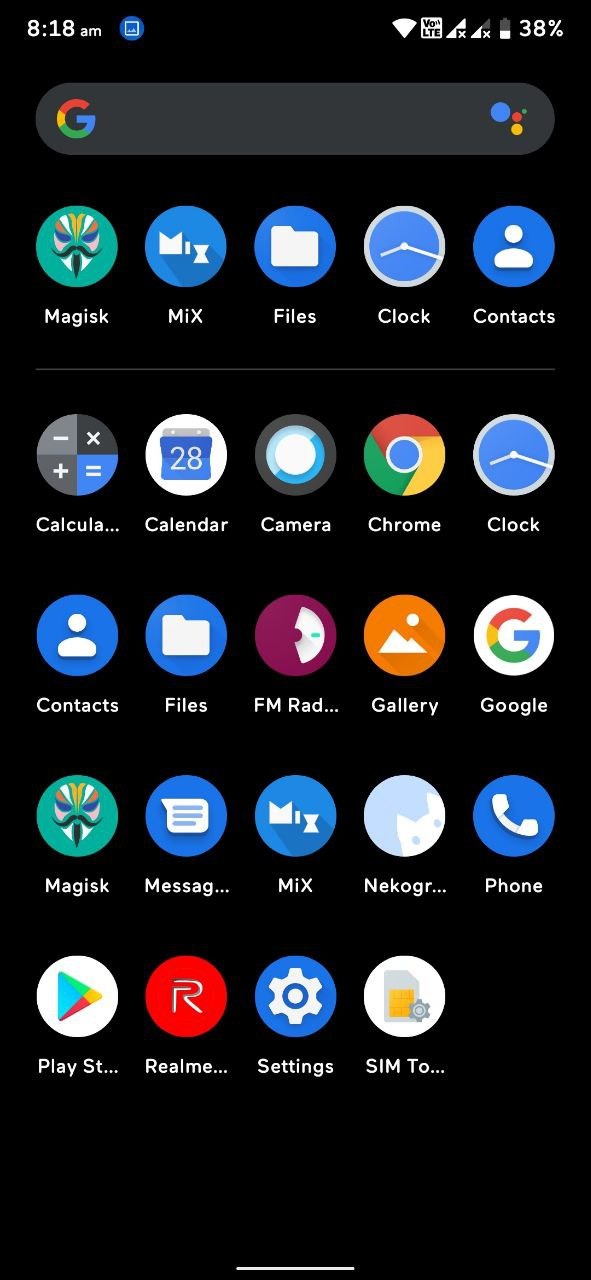Screenshot of a smartphone displaying the applications menu at 8:18 a.m. The device is in landscape mode with LTE enabled but showing no signal, indicating a likely disabled SIM card. The battery level is at 38%, and Wi-Fi is activated. At the top of the screen is a Google search bar with the standard "G" logo on the left.

The phone's background is black, enhancing the vibrant colors of the various app icons. The applications are arranged from left to right, in the following order: 

1. Magisk (featuring a Luchador mask icon)
2. Mix
3. Files
4. Clock
5. Contacts
6. Calculator
7. Calendar
8. Camera
9. Chrome
10. Clock (appears a second time)
11. Contacts (appears a second time)
12. Files (appears a second time)
13. FM Radio
14. Gallery
15. Google
16. Magisk (appears a second time with a Luchador mask icon)
17. Messages
18. Mix (appears a second time)
19. NekoGR
20. Phone
21. Play Store
22. Realme
23. Settings (depicted as a cogwheel)
24. SIM2 (indicating a SIM card manager)

Most of the icons maintain a standard blue background with the exception of unique icons for Magisk, FM Radio, Gallery, and Chrome. This comprehensive array showcases a typical app landing page with several duplicates, highlighting essential and some specialized applications on the user's device.